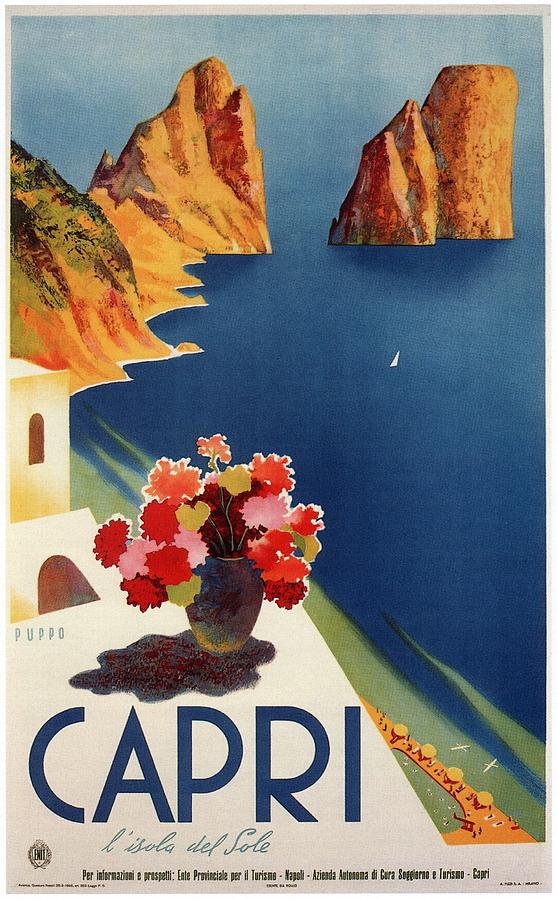This hand-painted advertisement for the island of Capri showcases a vibrant seaside scene. In the bottom left corner, the word "Capri" stands out in bold blue letters, with the cursive text "Del Sol" beneath it, suggesting a bright, sunny getaway. Above this text, a dark vase brimming with red, orange, green, and pink flowers casts a shadow on a white balcony surface. To the right of the vase, the serene blue water of the sea dominates the scene, interrupted only by a tiny white sailboat. On the left, a white building with oval windows and a strip of sand populated by beachgoers and yellow umbrellas draws the eye. In the background, four towering brown rock formations emerge from the sea, adding a majestic quality to this picturesque coastal landscape. The composition suggests a tranquil, inviting destination, perhaps intended to attract travelers.